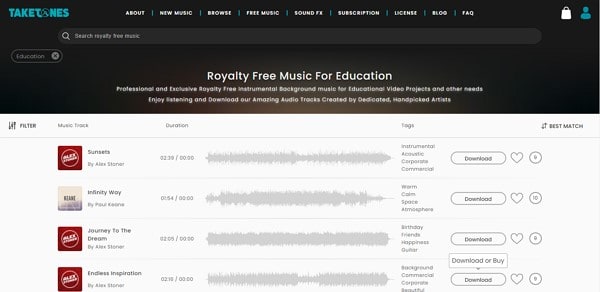A color screen capture from a computer monitor or laptop screen showcases a website. At the top, the website's name, "Take Tunes," is displayed in a lighter blue color. To the right, within a solid black horizontal rectangle, there are navigation options listed in white letters: "About," "New Music," "Browse," "Free Music," "Sound Effects," "Subscription," "License," "Blog," and "Frequently Asked Questions."

Below this menu, there is a search bar labeled "Search for royalty-free music." Further down, in white letters, the text reads: "Royalty-Free Music for Education." Accompanying this heading is a brief description: "Professional and exclusive royalty-free instrumental background music for educator video projects and other needs. Enjoy listening and download our amazing audio tracks created by dedicated handpicked artists."

Beneath this information, the capture shows three listed songs. For each song, the display includes the track name, the duration, relevant tags, and a "Best Match" indicator.